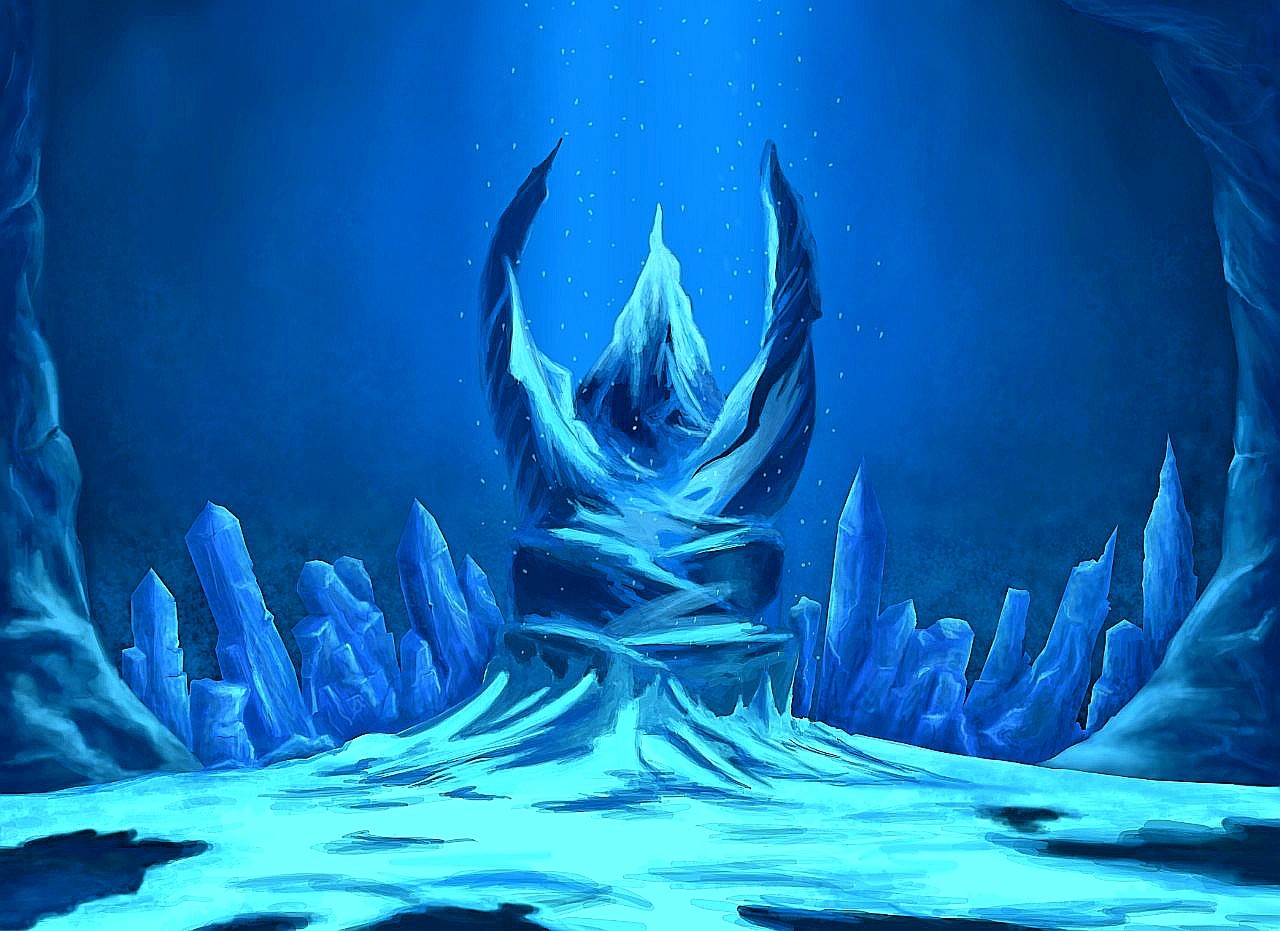This digital fantasy art illustration depicts an otherworldly, arctic-like landscape. Dominating the center of the scene is a throne-like structure, sculpted from jagged rock or crystal formations. The throne appears as a U-shaped pedestal, its rough, screw-like surface suggesting it might have erupted from the ground. A path reminiscent of a switchback mountain trail leads up to the throne, emphasizing its prominence. The throne itself emanates an ethereal light blue hue, possibly resembling flames or an electric aura, adding to its mystical appearance.

Surrounding the throne are dark blue crystals, their sharp forms jutting irregularly from the icy ground, hinting at a fantastical cavern environment. The lower part of the scene blends greenish-blue tones, with darker blue splotches adding depth and coldness. This surreal setting is lit from above, with a turquoise glow that bathes the entire throne area, enhancing the icy, otherworldly atmosphere. Small bubbles appear to rise from the ground, suggesting an underwater or submerged icy cave, lending an enigmatic quality to the artwork's setting.